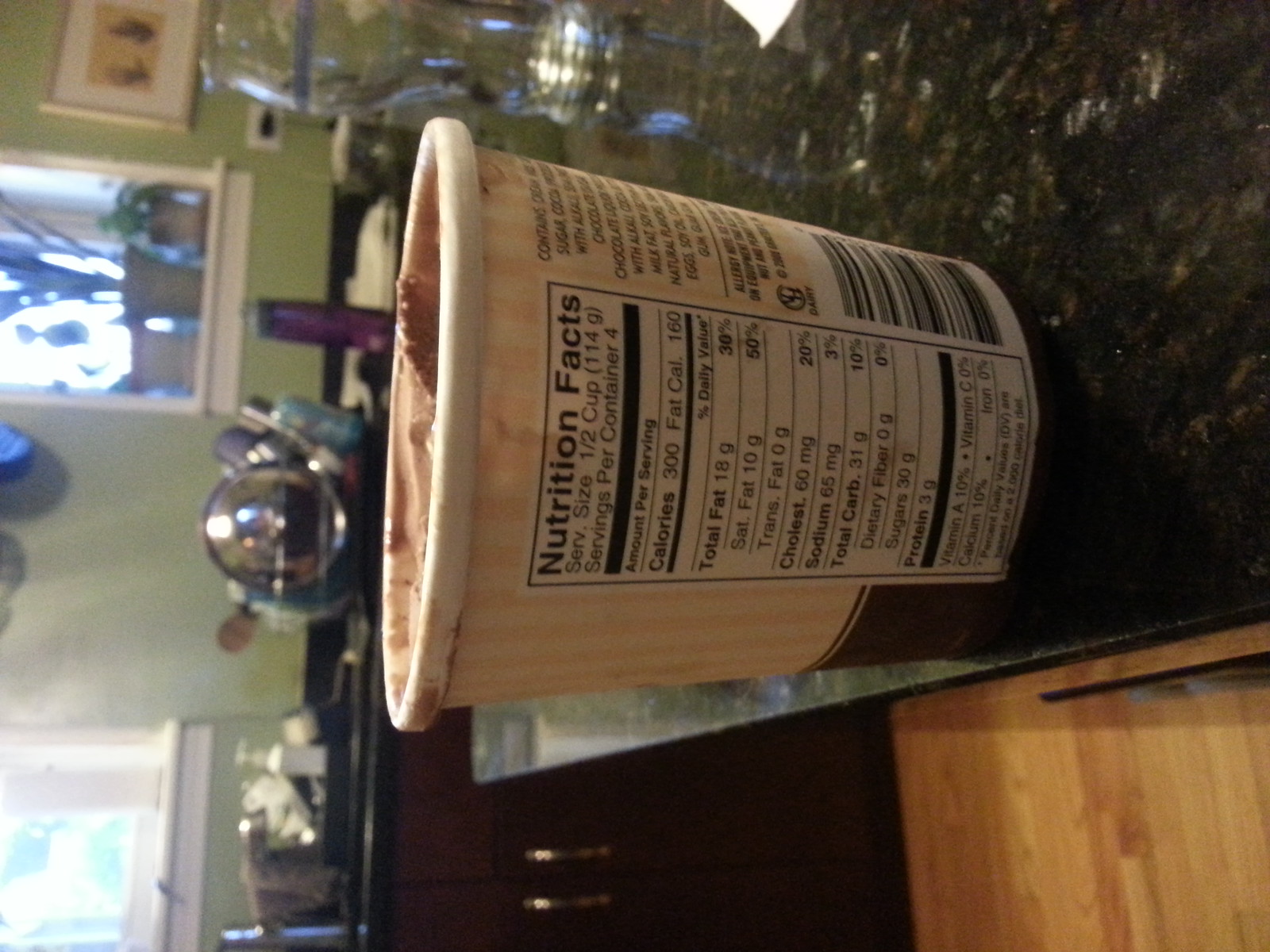In this image, we observe a sideways view of the back of an open ice cream container resting on a tabletop. To properly view the image, one would need to turn their head to the left. The container features nutrition facts on its back and has a dark brown base with white and yellow accents at the top. Adjacent to the ice cream container, at the bottom right corner, is a portion of a brown cutting board. The tabletop itself displays a reflective surface, showing hints of green, gray, and blue colors due to light beaming off it. However, the right side of the tabletop appears to be a darker black marble shade. In the background, two brown cabinets are visible along with a green kitchen wall that has two windows.